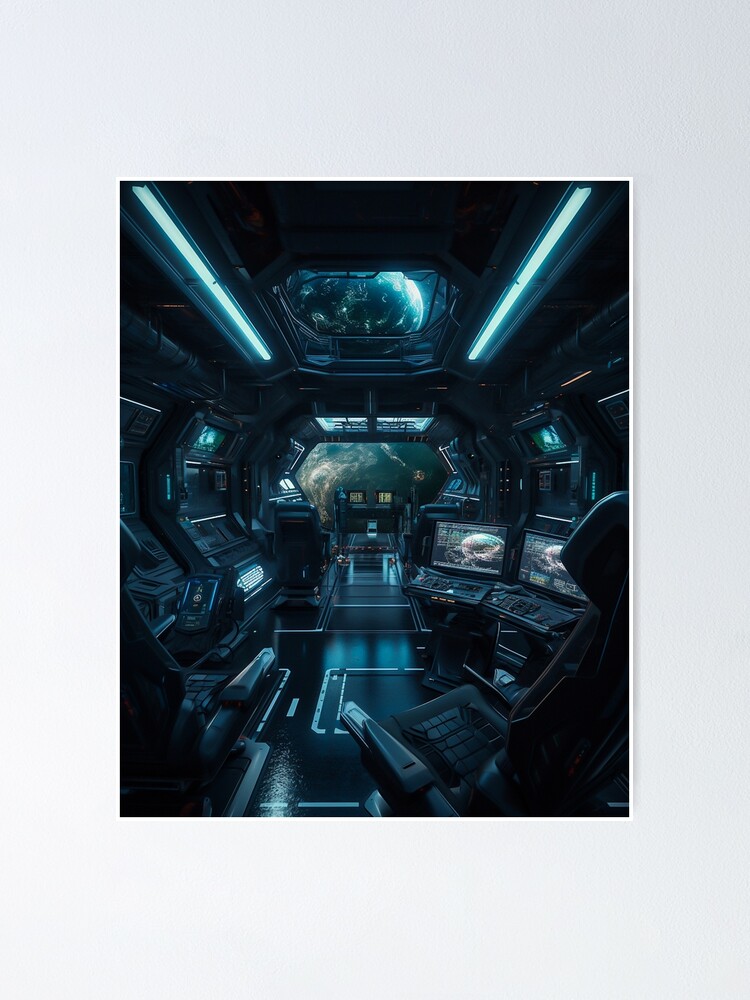This highly detailed sci-fi illustration portrays the interior of a futuristic spaceship, specifically the cockpit or bridge area. The scene is primarily colored in dark shades of black, gray, and dark blue, with a metallic, almost pristine aesthetic. The walls and floor are composed of dark, shiny materials that reflect light, adding to the clean, unused appearance.

At the front and top, hexagon and octagon-shaped view windows, respectively, offer breathtaking views of an Earth-like planet with blue oceans and white clouds, visible from high altitude or out of orbit. The ceiling of the spaceship is accented by bright blue fluorescent lighting bars that stretch across, casting a cool blue glow throughout the room.

Dominating the interior are numerous computer screens and consoles on the walls, all alive with glowing, though illegible, information. The left and right sides of the cockpit are filled with various panels, keypads, and buttons, indicative of advanced technology. The front also features additional control panels, contributing to the futuristic and highly equipped feel of the space.

Central to the room are two modernistic captain's chairs, often described as resembling gamer chairs, complemented by a couple of co-pilot or passenger seats. These chairs are positioned near the consoles, each fitted with armrests. One of the co-pilot seats even includes a tablet-like device mounted in a holder.

Overall, the image underscores a state-of-the-art, sci-fi technology ambience, with its glowing blue lights, sleek computer panels, and striking dual views of a distant planet, perfectly encapsulating the essence of an advanced spacefaring vessel.